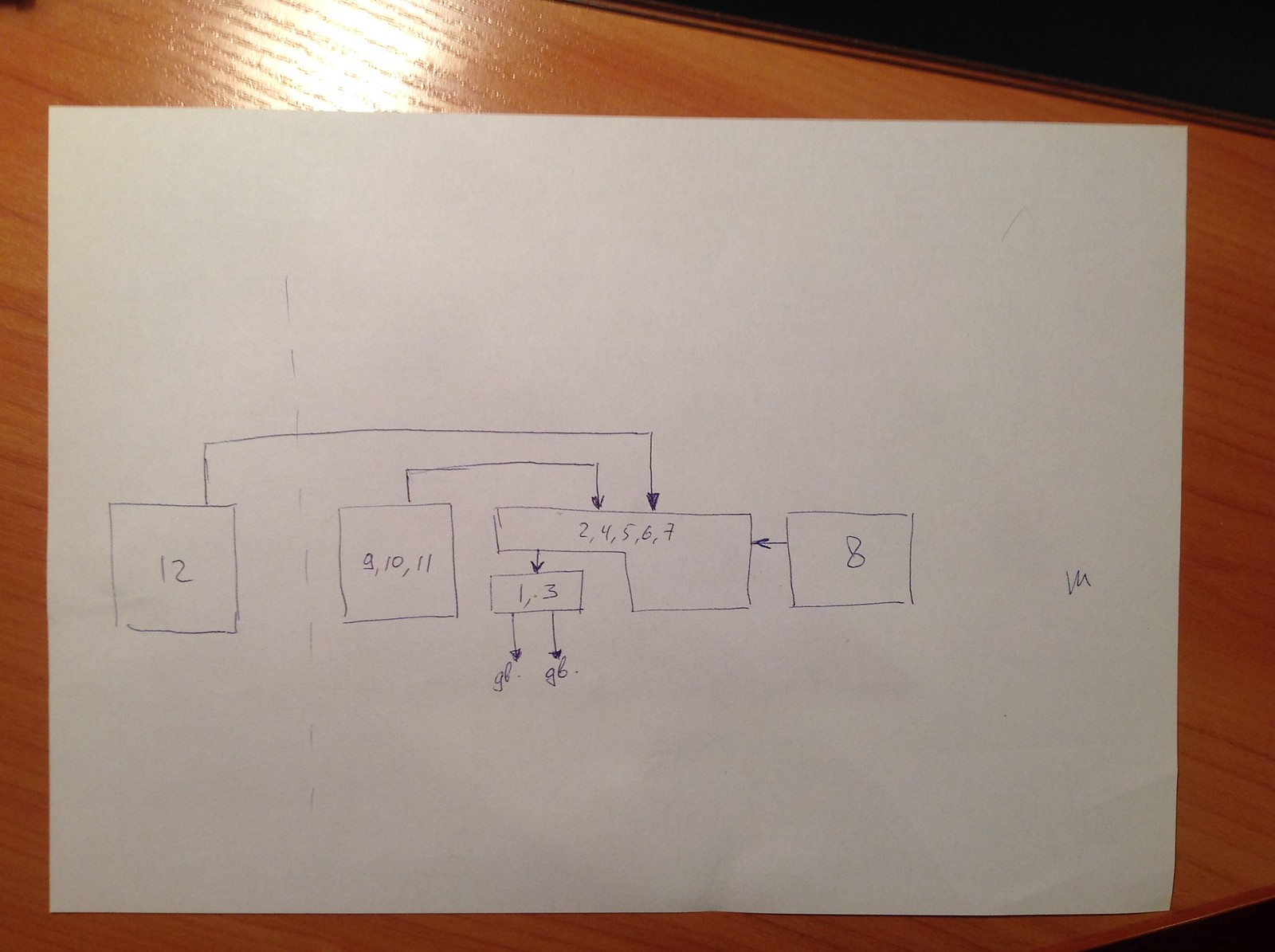The image features a light oak-colored, possibly laminate, wooden desk. Dominating the scene is a typical 8.5 by 11-inch white sheet of paper, oriented in landscape mode and occupying approximately 90% of the 4 by 6 photo frame. The paper contains a hand-drawn diagram resembling either a map or a complicated math equation. 

On the left-hand side, there is a neatly drawn square with the number "12" inside. From this square, a line with an arrow extends rightward, pointing to a more complex shape—a square with a tail—containing the numbers "2, 4, 5, 6, 7". Between these two shapes is another square marked with the numbers "8, 10, 11". Below this intermediary square is a small rectangle labeled with the numbers "1 and 3". On the far right side of the paper is another square, plainly labeled with the number "8". The layout of the diagram suggests it could be either a conceptual map or a mathematical flowchart.